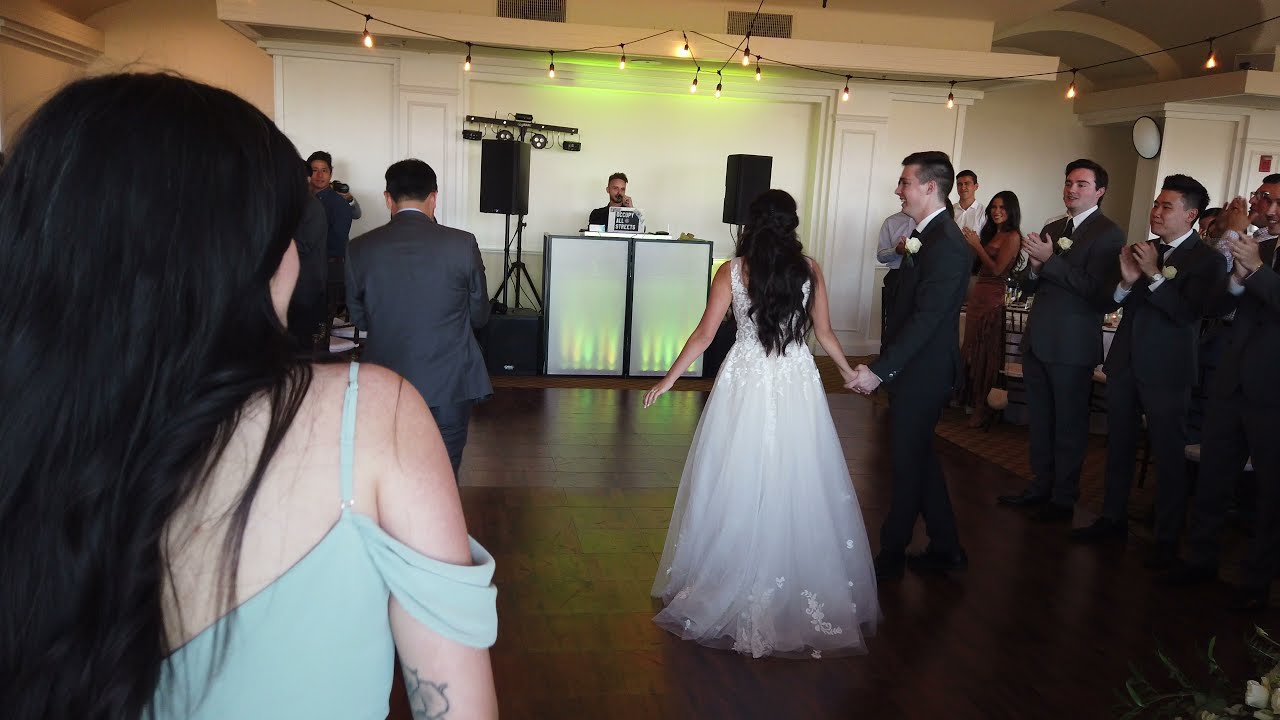In the center of a large wedding hall with white walls and wooden paneled flooring, a bride and groom are captured at the forefront of the image, surrounded by guests. The bride, a Caucasian woman with long black hair, is dressed in a sleeveless, lacy white gown adorned with floral frills. She stands with her back to the camera, holding the hand of the groom—also Caucasian—who faces her in a black suit and short dark hair. They appear to be on the dance floor, perhaps having just shared their first dance. To the far end of the room, a DJ booth set against a white wall with pillars is visible, featuring two large speaker stands and illuminated rectangular panels. The DJ, a Caucasian man with short dark hair, works from a laptop, providing the celebratory music for the event. Surrounding the couple are numerous guests, with a notable woman in a blue gown positioned to the left side of the frame. Scattered around the space, several groomsmen in matching suits dot the scene, adding to the joyous, lively atmosphere of the wedding celebration.